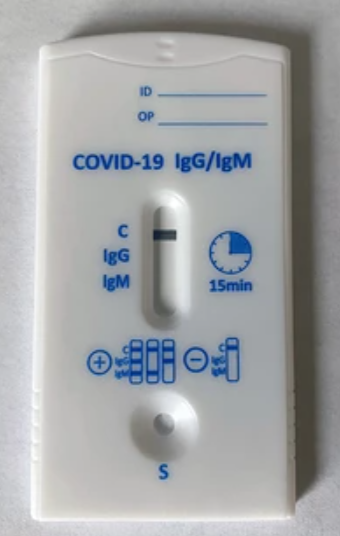This vertical photograph captures a detailed view of a COVID-19 rapid test kit. The kit itself is a rectangular, white plastic device featuring a circular sample opening at the bottom and a long, capsule-like depression in the center for displaying test results. The inscriptions on the device are printed in blue. 

In the upper right-hand section of the tester, there is an ID line, and directly below it, an OP line. The title "COVID-19 IgG/IgM" is prominently displayed in a blue font across the area just above the results window. To the left of the results window, there are labeled lines: 'C' for control, 'IgG' for Immunoglobulin G, and 'IgM' for Immunoglobulin M.

Also featured is a clock icon accompanied by the label "15 MIN," indicating that this is a 15-minute rapid test kit. Directly below the results window and above the circular sample opening, there are illustrations of possible line combinations that designate positive and negative results. A positive result is shown by any combination of three lines (at the top, middle, and bottom positions of the results window), while a negative result is indicated by a single line at the control position.

The sample opening is marked with a blue 'S' at the 6 o'clock position at the bottom. The entire test kit is set against a clean, white background, highlighting its features and functionality.